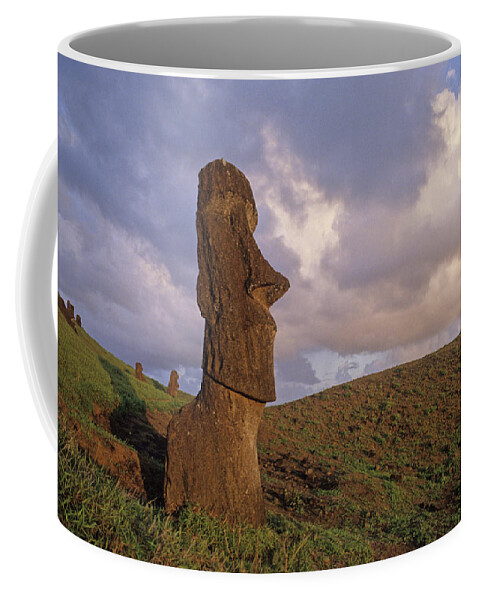The image primarily features a close-up view of a standard-sized coffee mug, which takes up almost the entire frame. The mug is adorned with an intricate depiction of Easter Island heads, or moai, showcasing their chiseled faces, noses, mouths, and jawlines in a striking brown and goldish-rusty color. The foreground Easter Island head is set against a green, hilly landscape with patches of exposed brown dirt. In the background, several more moai can be seen, though they are slightly blurred due to their distance. The sky overhead is a grayish-blue, heavily clouded, but with some sunlight piercing through the center of the cloud cover on the right side of the central moai, casting shadowy effects below. The overall scene suggests overcast weather, hinting at potential rain. The statues appear well-preserved, with no visible signs of wear or damage.